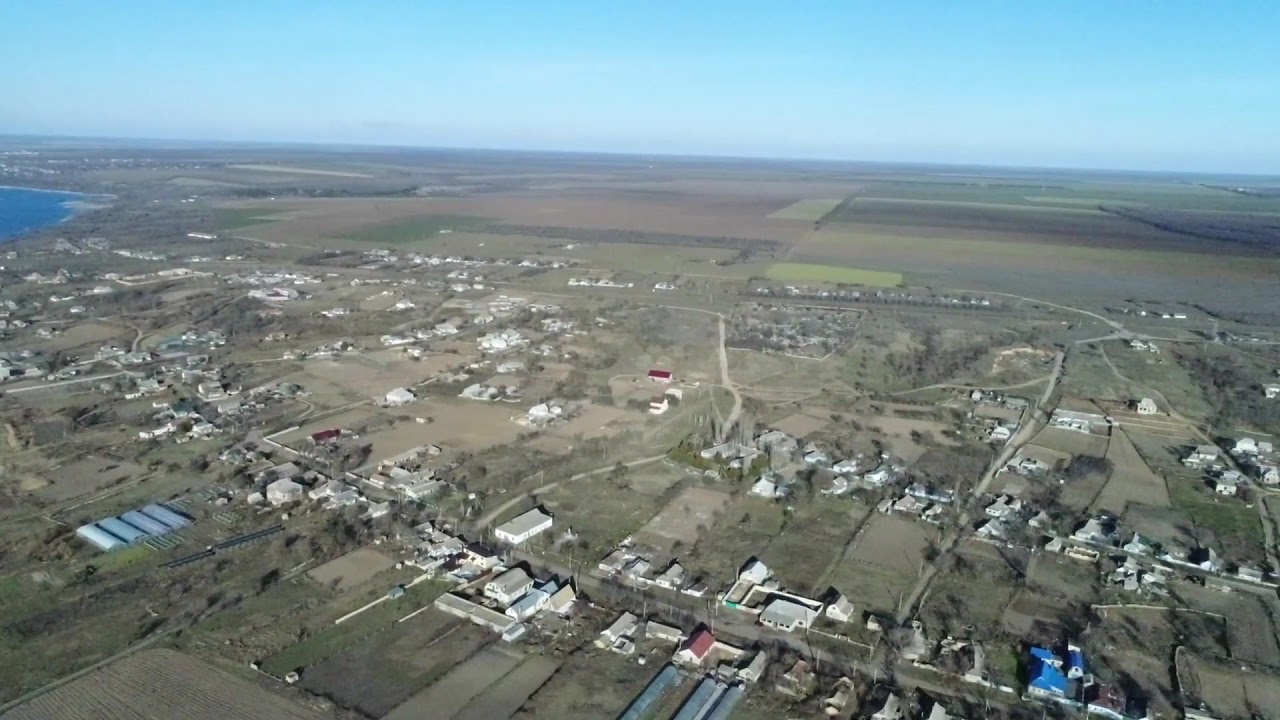This aerial photograph, taken from high above, captures a sunlit, semi-hazy landscape featuring an industrial and residential mix. In the foreground, a small town is visible with a network of streets and driveways connecting various buildings, including residential homes with distinctive blue and red roofs and larger industrial structures resembling Quonset huts. Telephone poles line the streets, and fences enclose some properties. Leafless trees dot the scene, adding to the desolate feel. Extending beyond the town, the flat terrain transforms into a patchwork of green and brown agricultural fields spreading to the horizon. The horizon itself appears hazy, with a clear blue sky above indicating a daytime setting. In the upper left corner, part of a body of water intrudes into the frame, adding a touch of natural beauty to the predominantly developed landscape.